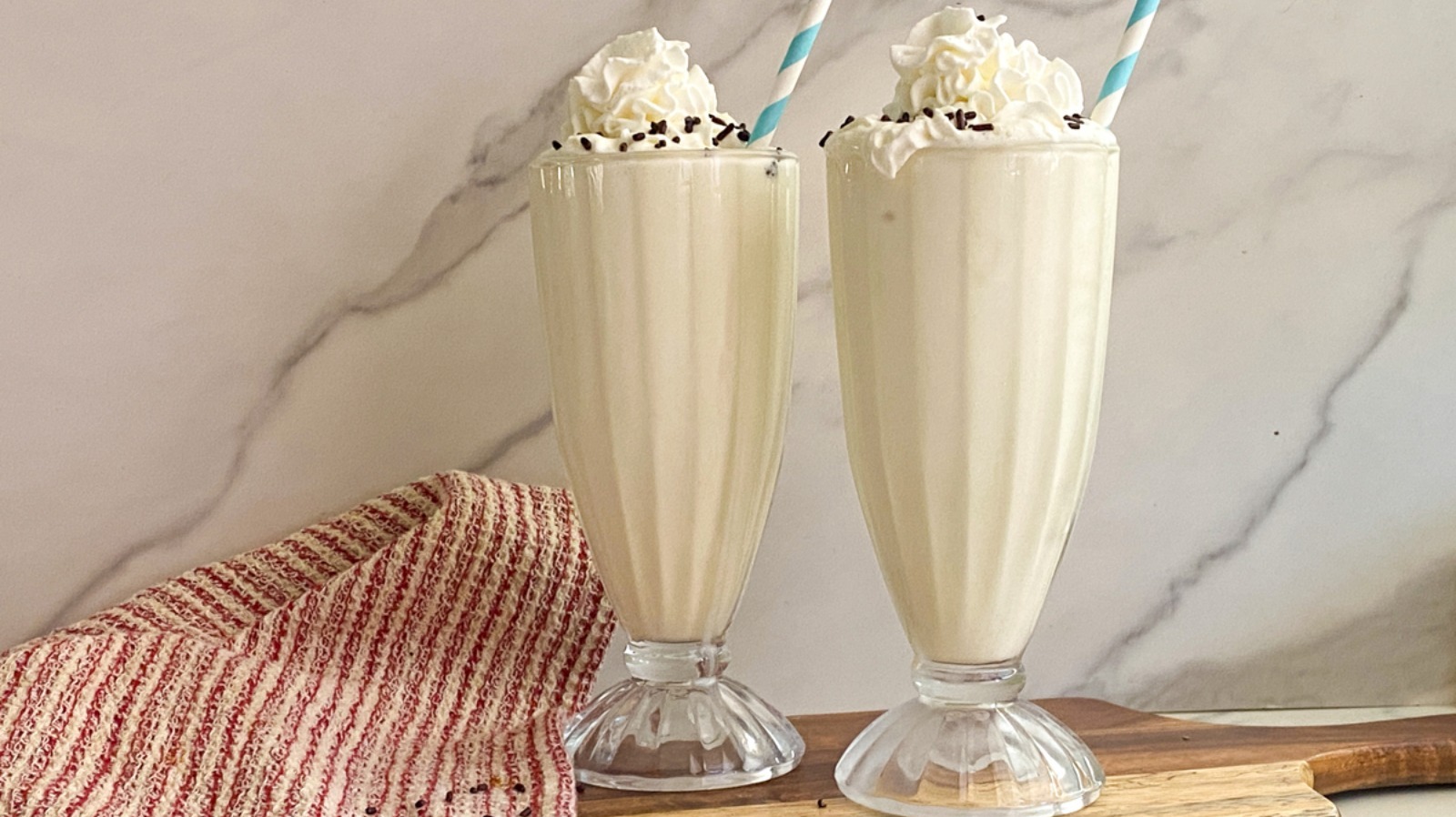The photograph showcases two tall, ornate milkshake glasses, the kind typically found at a vintage soda fountain. Each glass is filled with what appears to be creamy vanilla milkshakes, topped with off-white whipped cream arranged to mimic flower petals. Garnished with small black chocolate sprinkles, the milkshakes have a nostalgic charm accentuated by the blue and white striped paper straws sticking out of them. The glasses, with their narrow necks and fluted bases, are resting on a light brown wooden cutting board with a handle. To the left of the glasses, there is a red and white striped cloth, adding a pop of color against the white and gray marbled backdrop. The overall setting exudes a classic, retro vibe.